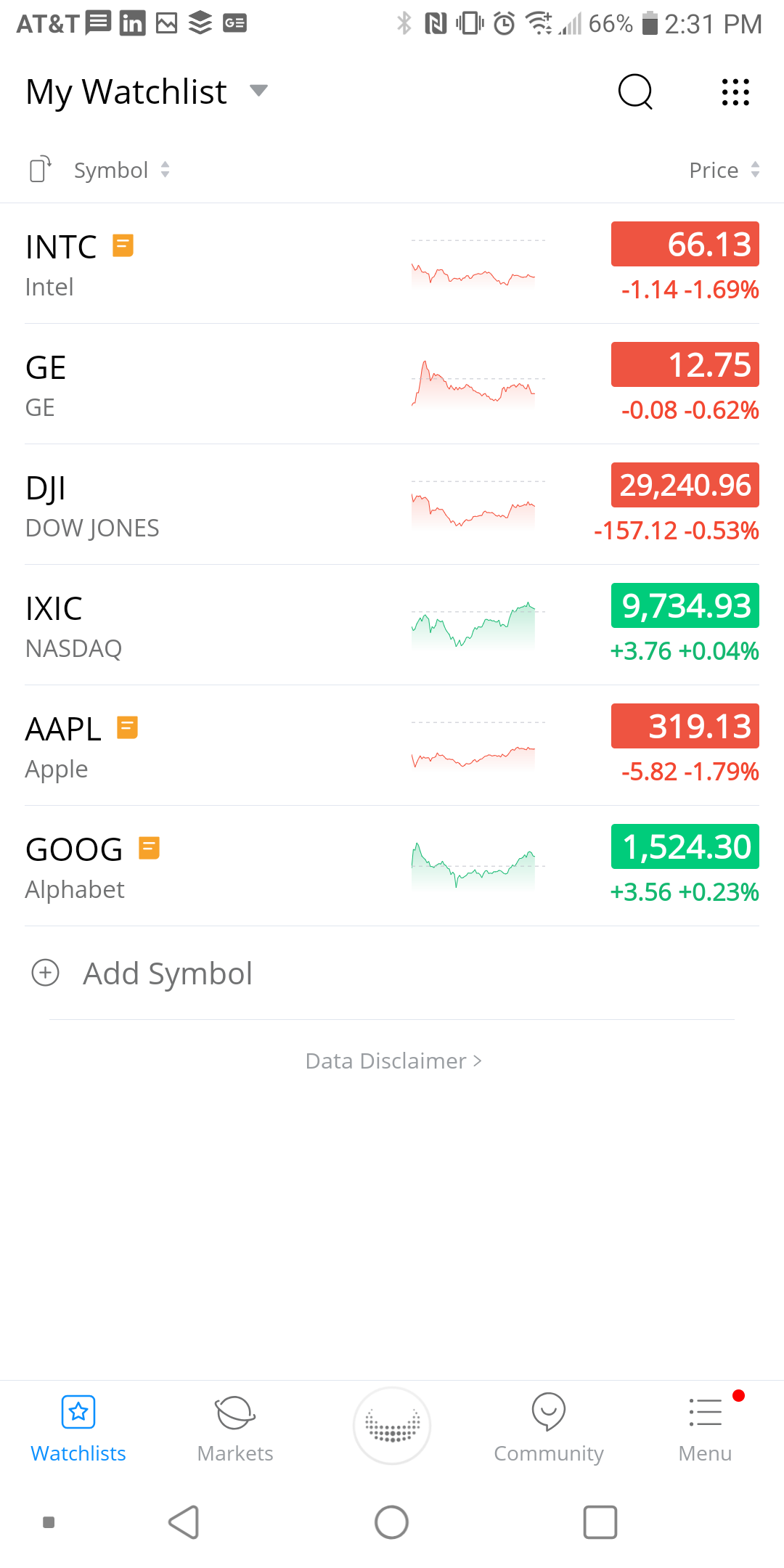The image is a screenshot of a smartphone displaying a stock market tracking app. In the top left corner, the network carrier is AT&T, and adjacent to it on the right, the time is shown as 2:31 p.m. The phone’s battery life is at 66%, and there is a strong Wi-Fi connection. 

The main section of the screen features a section titled "My Watch List," which lists six stocks: INTC (Intel), GE (General Electric), Dow Jones, NASDAQ, Apple, and Alphabet. 

Each stock's performance is indicated next to its name with colored numbers: red for losses and green for gains. Between the stock names and their performance metrics, there are small line graphs, providing a quick visual representation of each stock’s price movement. 

Overall, the screenshot clearly depicts the user monitoring the stock market via a mobile app, observing real-time changes in their selected stocks’ performances.